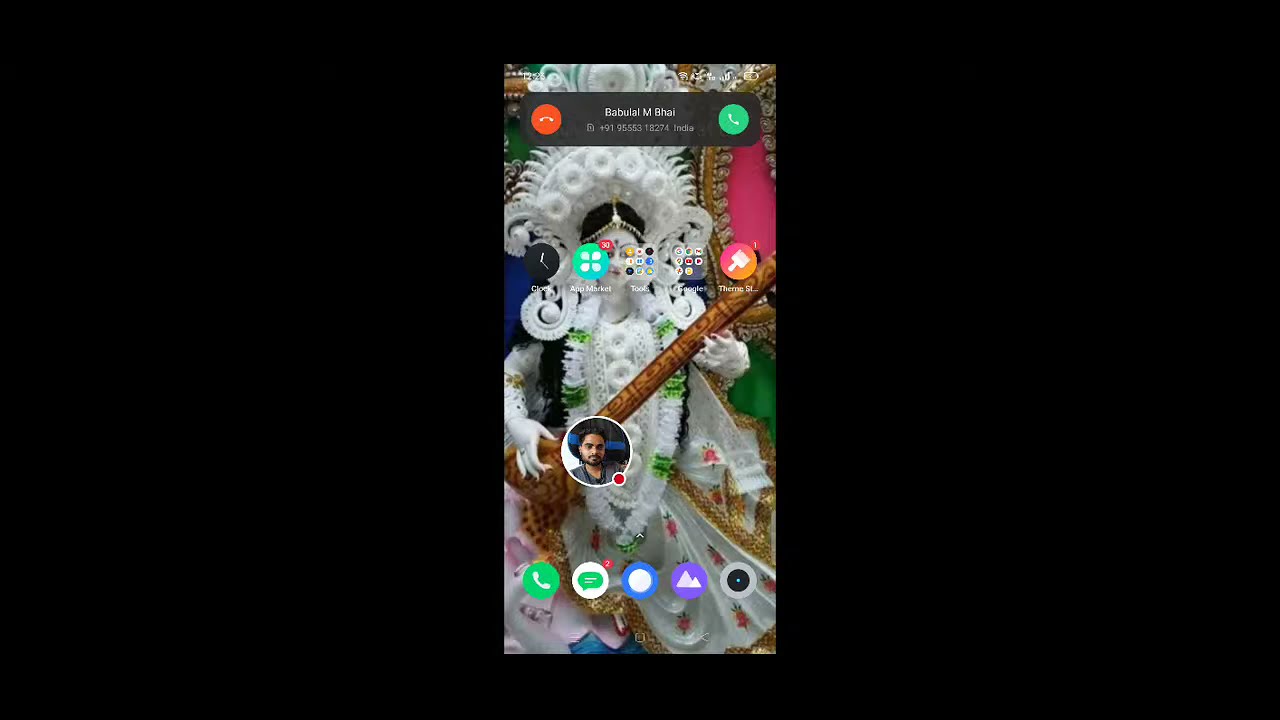The image appears to be a screenshot from a cell phone, showcasing an intricate wallpaper depicting a statue or representation of a Hindu goddess, possibly Saraswati, often associated with wisdom and music. The figure is adorned in an elaborate white costume with a meticulously carved white cascading crown that extends below her shoulders. Her face is painted white, accentuated by a small black dot on her forehead (a bindi), and she wears a gold chain encircling the top of her hair. She holds a sitar, a long musical instrument reminiscent of a guitar in structure but much longer, emphasizing the cultural and artistic background. Also visible on the screen are various icons for applications, indicating it’s likely a Samsung phone, and at the top, a notification of an incoming call from a contact named Babula M. Bai, with the region specified as India. This notification includes the standard red and green phone symbols to decline or answer the call, respectively, with a circular avatar of a young Indian man with a beard and mustache displayed in the center. Additional icons at the bottom imply functionalities for calling or web surfing.